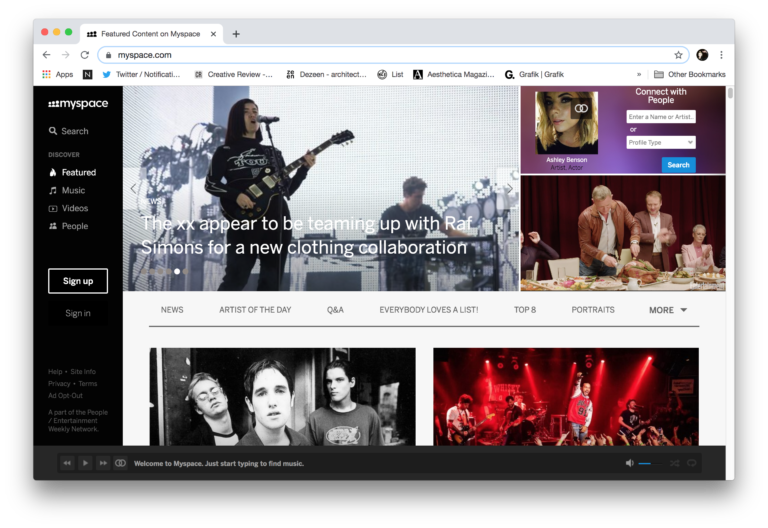This screenshot captures an open Chrome tab featuring the Myspace homepage. At the top of the tab, it reads "Featured Content on Myspace." The Chrome bookmark bar is visible, showcasing bookmarks for Twitter, Dezeen, and Aesthetica Magazine. The main content displayed on the Myspace page includes various news articles and advertisements.

Prominently featured is a news article with a picture of a white man with long black hair, dressed in a black t-shirt and pants. He is holding a black electric guitar and singing into a microphone. Beneath the image, a headline in white font announces that The XX are teaming up with Raf Simons for a new clothing collaboration.

To the right, there is an advertisement encouraging users to "Connect with people in your area" with a prompt to "Enter your name here."

Below, another photo displays elderly white people carving a turkey. Further down the page, a white bar with gray text lists sections titled "News," "Artists of the Day," "Q&A," "Everybody Loves the List," "Top Eight," "Portraits," and more.